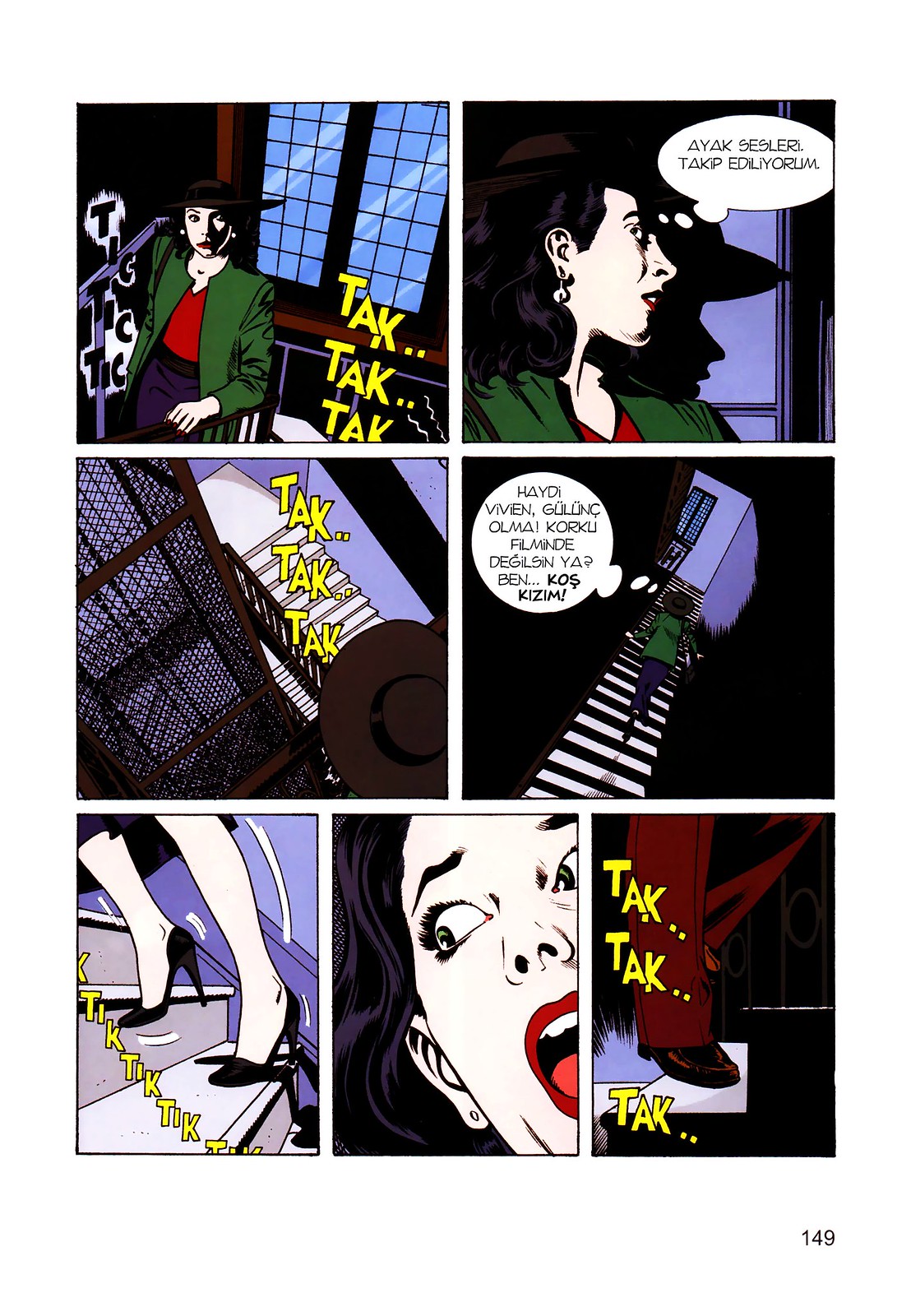The comic strip features a series of seven colorful panels divided into three rows. The top row consists of two panels: in the first, a woman with dark hair wearing a green jacket, red blouse, blue pants, and a black hat stands before a window latticed with grids. The caption features onomatopoeic sounds, "TIC TIC TIC," alongside "TAC TAC TAC." The second top panel shows the woman from her right profile, appearing to speak as indicated by quotation marks emanating from her head, likely in another language. 

The middle row contains two panels, with the first depicting urban scenery, including a white building and a black fence. The "TAC TAC TAC" sound reappears in this panel along with another quotation in a foreign language. In the second middle panel, the woman ascends a staircase toward a blue door, the "TIC TIC TIC" sound continuing, marking her heel clicks.

In the bottom row, the first panel narrows in on the woman’s legs and high heels as she moves upstairs. The center bottom panel captures her distressed face, mouth open in a scream, highlighted with red lipstick and a vivid red tongue. The final panel in the bottom row shows a man's leg clad in brown pants and dark shoes descending the stairs, accompanied again by the "TAC TAC TAC" noise. The sequence suggests a tension-filled moment as the woman reacts with fear to the approaching figure.